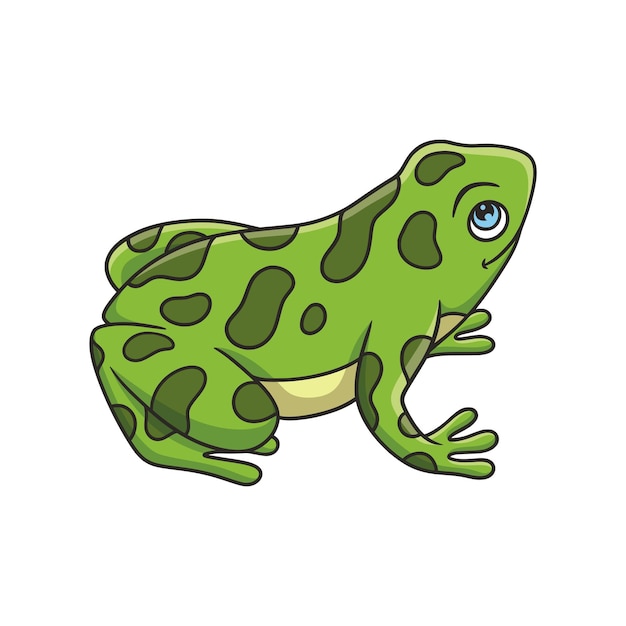This image is a simple, cartoon-like illustration of a green frog with a smooth, rounded body and distinctive darker green spots. The frog is shown in a crouching position with all four of its webbed feet firmly planted on the ground. Its underbelly is a light yellow color. One of the frog's most striking features is its blue eye, which stands out against its green body. The illustration includes a slight smile and an eyebrow, giving the frog a friendly expression. The background of the image is plain white, providing a clear contrast to the frog's vivid colors and dark green outlines. The image accurately captures a side view of the frog, showcasing its detailed markings and simple design.